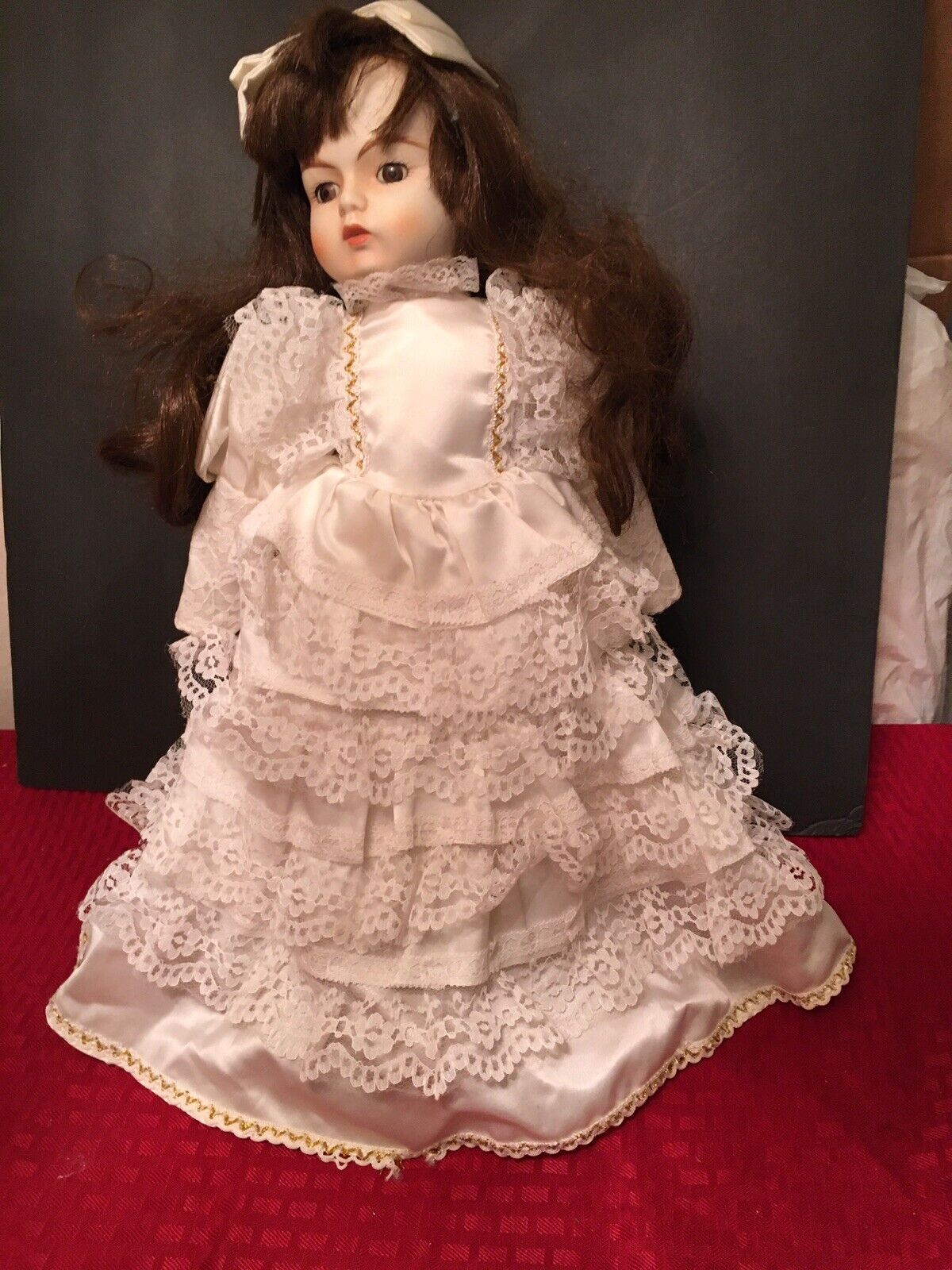This image depicts an old porcelain-faced Victorian-style doll standing upright. She is adorned in a very frilly, multi-layered white dress with intricate gold stitching along the bottom and down the sides of the chest. The dress, featuring satin and lace with numerous ruffles, is complemented by lace around her neck. Her long, curly brown hair is topped with a matching white bow or ribbon. The doll has big dark brown eyes, light brown eyelashes, bright red cheeks with two pink spots, and vibrant pink lips, enhancing her pale complexion. She stands propped up against a dark gray or black background, positioned on a bright red cloth that possibly has an iridescent design. This intricate and well-preserved doll appears to be a valuable collector's item.